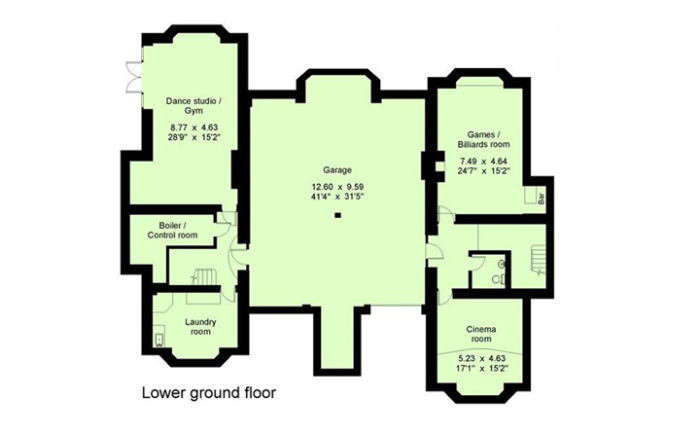Title: Detailed Floor Plan - Lower Ground Floor

Description:

This detailed schematic floor plan represents the lower ground floor of a building, such as one might find in a hotel with fire escape routes clearly marked. The layout is artistically presented with thick black lines defining the outer walls, and thin black lines delineating doorways and interior spaces. The overall color scheme inside the rooms is a light green, enhancing the visual clarity of each designated area.

- **Central Area:** The central portion of the floor layout is labeled "Garage," and is prominently measured to specify its dimensions.
  
- **Top Left Corner:** This section houses a "Dance Studio/Gym," with specified measurements. It features both exterior and interior doorways, providing accessibility.

- **Adjacent Areas:**
  - A "Boiler Control Room" is situated next to a staircase, complete with its own doors leading into the dance studio, garage, and additional spaces.
  - There is a "Laundry Room" positioned at the bottom section near the garage.

- **Top Right Corner:** This area is dedicated to a "Game/Billiards Room," also clearly measured. Adjacent to it is a small washroom, likely another interior doorway leading towards unidentified areas.

- **Bottom Right Corner:** 
  - A "Square-Shaped Room" shows typical half-bath fixtures, including a toilet and sink, and connected to an interior door leading towards the garage.
  - Below this section lies a "Cinema Room," complete with its measurements and indicated with window placements for natural light.

- Throughout the layout, several staircases and washroom indicators are noted, ensuring functional connectivity between different areas.

This meticulously detailed floor plan provides a comprehensive overview of the lower ground floor’s layout, useful for navigation, planning, and safety purposes.